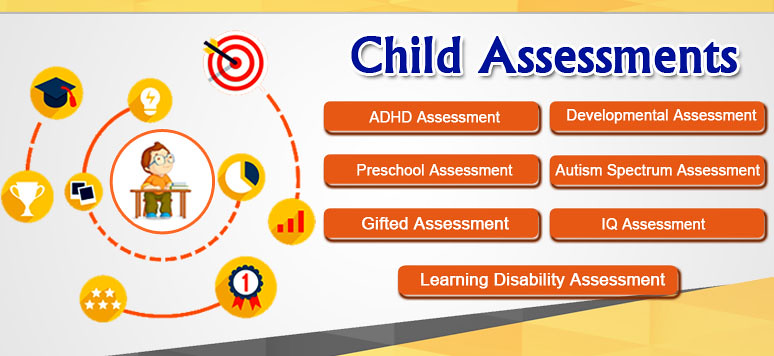This detailed color graphic features a white and yellow background with complementary orange elements and blue text. The right side prominently displays the title "Child Assessments" in blue, followed by a series of orange rectangular boxes with white text that list the types of assessments: ADHD Assessment, Developmental Assessment, Preschool Assessment, Autism Spectrum Assessment, Gifted Assessment, IQ Assessment, and Learning Disability Assessment. 

On the left side, a stylized cartoon-like depiction of a small child sitting at a brown desk is central. The child, wearing an orange shirt, brown pants, blue shoes, and glasses, looks to the top right at a target with an arrow in its bullseye. Surrounding the child are three concentric rings, reminiscent of atomic models. Each ring connects various clip art images: a light bulb at the top, photos to the left, a pie chart to the right, and moving outward, a graduation cap with a red tassel, a trophy, five stars, a number one blue ribbon, and a bar chart, all linked together in a network of dashed and solid lines, providing a visual representation of the different aspects of child development and achievement.